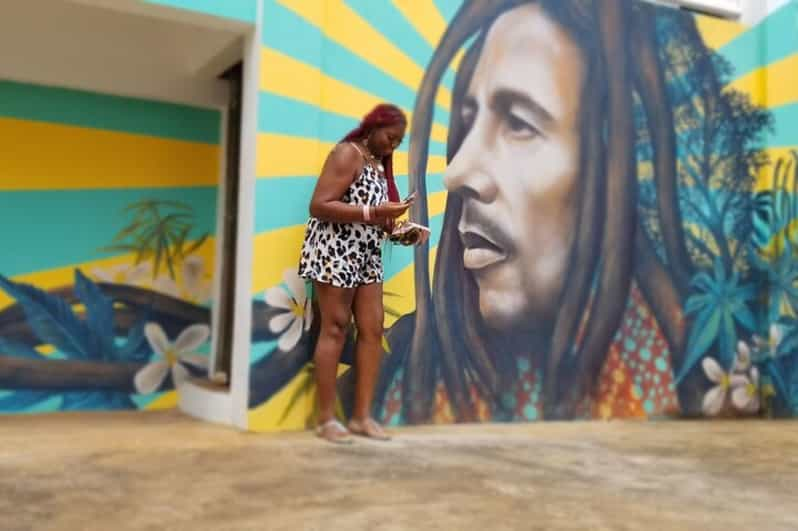The image captures a one-story building adorned with a vibrant mural of Bob Marley. He stands in profile, his dreadlocks cascading down, wearing a turquoise and orange tropical shirt. Sun rays in yellow and turquoise emerge behind his head, set against a blue background filled with white plumeria flowers and lush tropical foliage. In front of the mural, a black woman with red braided hair stands looking down at her phone. She is more sharply focused than the mural and wears a leopard-patterned white short set. Despite some aspects of the image being out of focus, the details of the mural and the woman's attire are vivid and clear, suggesting a blend of urban artistry and everyday life.